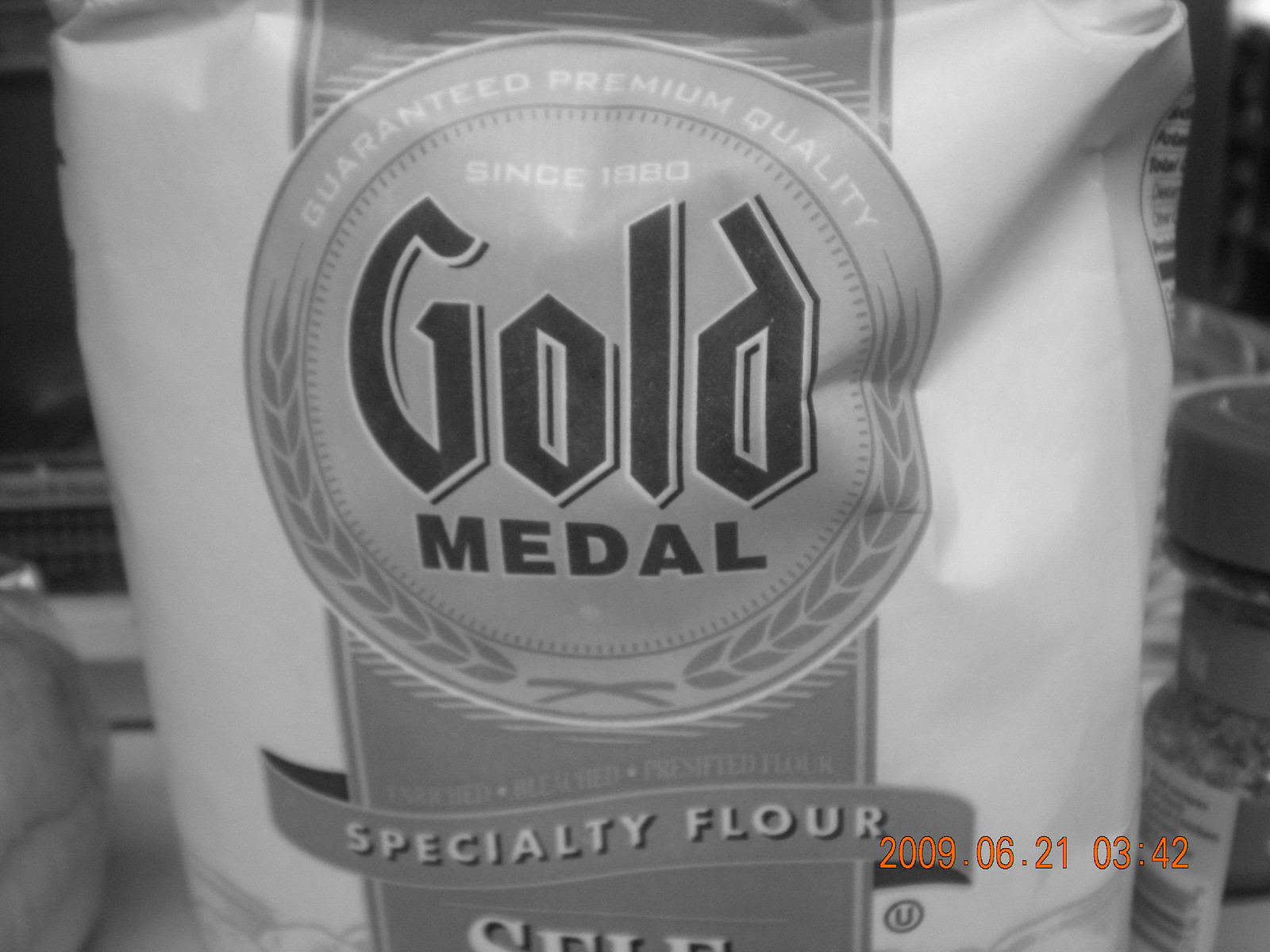This black-and-white photo captures a close-up view of a somewhat crinkled bag of flour, potentially taken in a grocery store or convenience store with minimal lighting, suggested by the greyed-out appearance. The bag is predominantly light in color with a contrasting darker band running vertically down the center. Prominently displayed in the middle of this band is a large circular emblem with the dark text "GOLD MEDAL." Above this, white text reads "GUARANTEED PREMIUM QUALITY SINCE 1880." Below the emblem, within a ribbon banner, more white text states "SPECIALTY FLOUR." The photo has a timestamp in the bottom right, indicating it was taken at 03:42 on June 24, 2009. Possible hints of other items, such as seasoning and buns, appear at the edges but are unclear due to cropping.